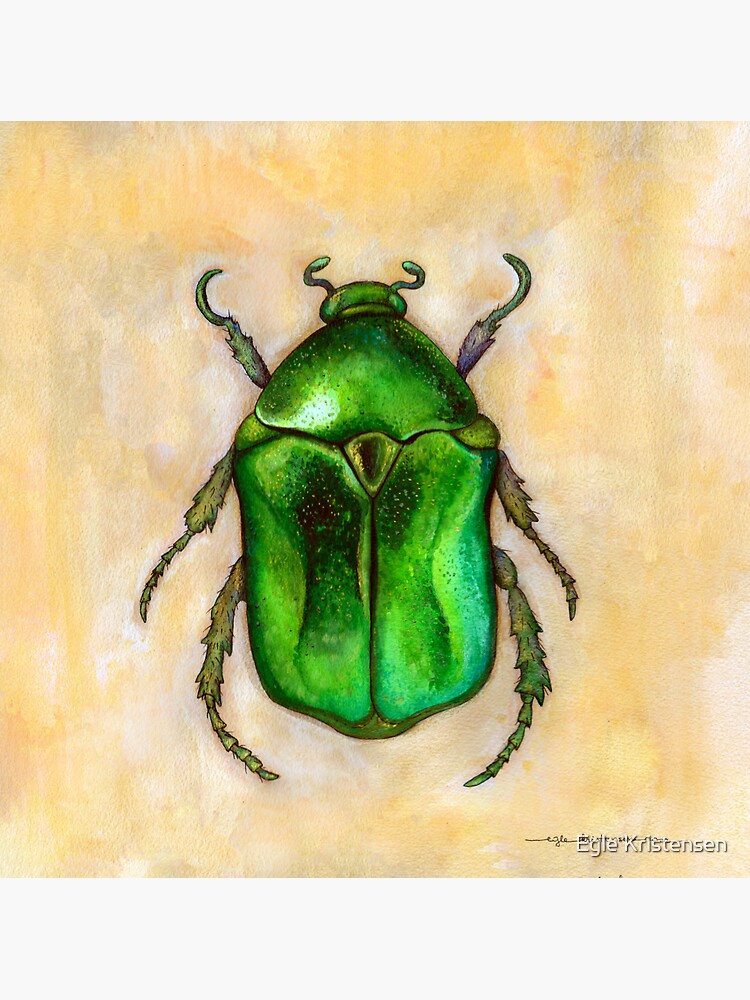The image features a detailed, close-up illustration of a beetle set against a tan background with hues of yellow and white. The beetle, primarily light green with dark green accents, prominently displays its six creepy, hairy legs and its neon green head from which two light green antennae protrude. The beetle's segmented body is clearly depicted in three parts, each resembling a shell, with shades transitioning from dark to light green. The legs, four pointing downwards and two curving towards the head, even show hints of violet. The bottom right corner of the image bears the printed name "Eagle Christensen," presumably the artist, who added a handwritten signature beside it. Overall, the beetle has a strong, armored appearance, lending an almost lifelike quality to this striking specimen illustration.